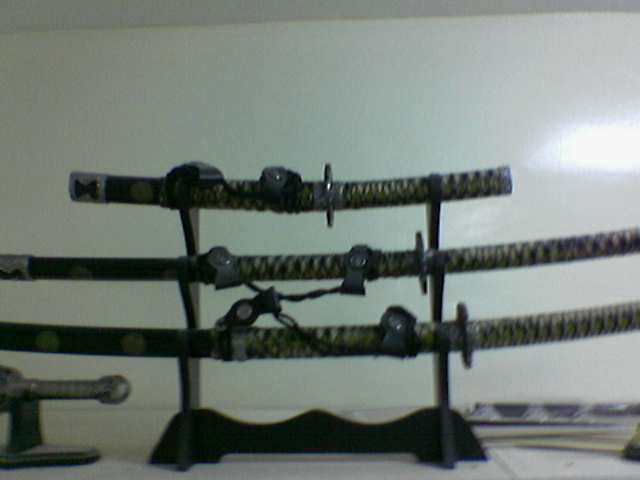This detailed indoor photograph, taken against a pure white background, showcases an intricately designed black sword stand holding three Japanese swords arranged horizontally. The stand, which includes three vertical sections, supports the sheathed swords, each one featuring a combination of black and tan twine wrapping. The bottom sword is the longest, followed by a slightly shorter one in the middle, and the shortest sword on top. Each sword handle, extending out of the frame, is dark in color. The stand's top section also holds a fourth weapon, possibly a dagger, approximately 18 inches long, displayed prominently with a black 'M' shaped symbol on the left-hand side of its silver hilt. The lighting in the image is dim, causing a slight blur and a hint of reflection that suggests it was taken indoors, with some light shining from a ceiling fixture, likely contributing to the flash visible in the upper right corner.